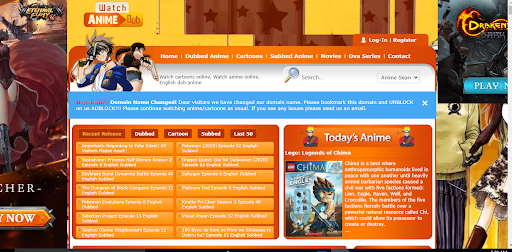This screenshot appears to be of a video game interface, possibly showcasing an anime-themed game. Starting from the left side, a character with partly visible red and red-yellow hair is noticeable. The text "Eternal Play" is displayed in the bottom left corner. Adjacent to this, there is an orange tab partially off the left side with visible white letters "TR" above it.

On the right side, the scene looks like an outdoor setting with a dragon sitting in the middle of a road. Underneath the dragon, the text "Red Dragon" is written in black, darkened by a shadow. To the right, there is a blue tab with the word "Play" in white, half visible off the side of the screen.

In the middle-right section, two anime characters are partially visible from the chest down. One character wears a yellow shirt with blue-black pants, while the other dons a red shirt with long brown hair and a skirt adorned with a floral pattern.

At the top left corner, a white tab with red text reads "Watch," and below it, 'Anime Dub' is written in white and red. Beneath these are red and yellow tabs depicting two anime characters. To the right of these tabs, six clickable white lettered tabs are positioned sequentially, with "Register" and "Log In" situated above them.

A white space with some information occupies the document's right side, featuring a search bar and a thin blue bar about an inch wide with white lettering. Below this, towards the left side, about one-third over and beyond to the white area, there's a dark orange border containing eight orange rectangles with white letters arranged in pairs. Adjacent are five red tabs, the first with yellow lettering and the remaining four in white.

Moreover, on the right side, an anime character with blonde hair is labeled "Today's Anime," followed by another image of the same character. Beneath this, partial text "Legends of" is discernible, followed by the image of a video game and additional information presented in white letters.